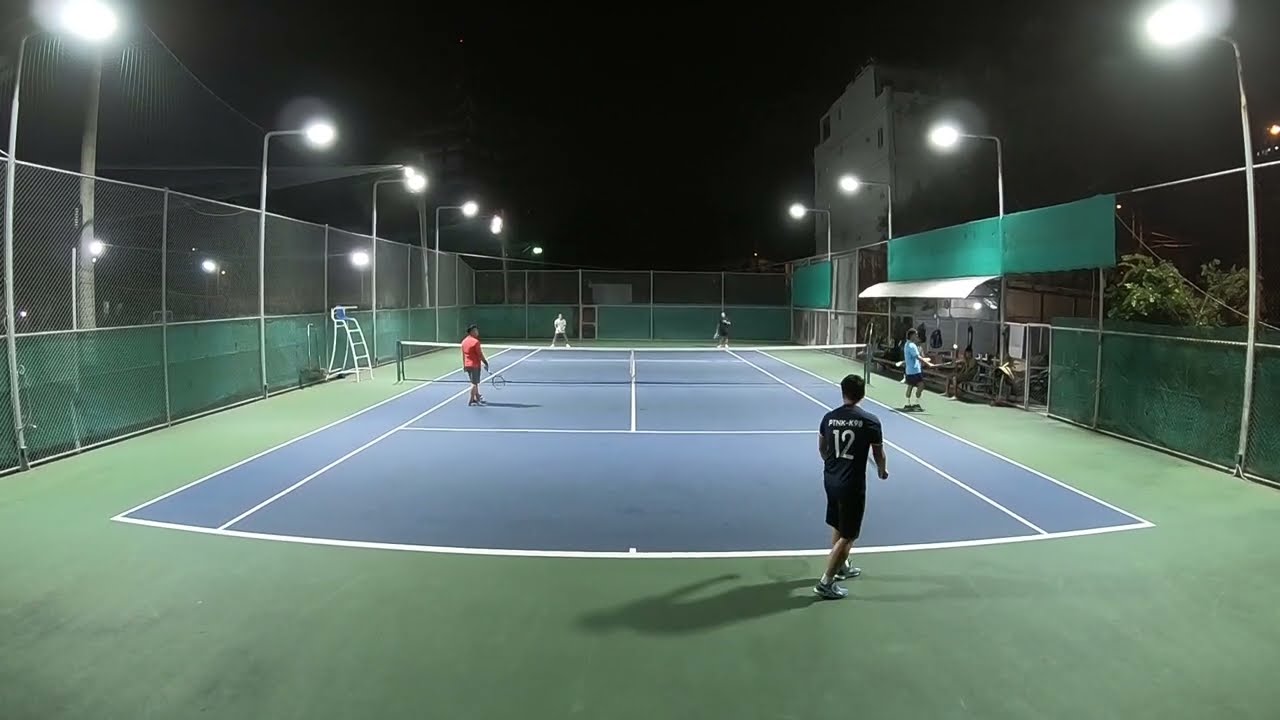The photograph captures an outdoor tennis court under the night sky, brightly illuminated by overhead lights. The court itself is entirely blue with white lines marking the various areas of play, and it is surrounded by a tall chain-link fence, most of which is covered at the bottom with a see-through green canvas. There are five people present: four players actively engaged in a tennis match, and one person observing from the side. In the foreground, closest to the camera, a player is wearing black shorts and a black shirt emblazoned with the number 12. To the right side of the court stands an onlooker in a blue t-shirt and black shorts. Meanwhile, another player in a red t-shirt and gray shorts, holding a tennis racket in their right hand, is positioned closer to the net. The edges of the court are solid green, contrasting with the blue playing surface. To the right, there is a towering three-story building visible in the background. The top of the fence features lights that shine down onto the court, ensuring clear visibility for the ongoing night match. Also on the left side, a small referee stand can be noted, adding a professional touch to the setting.